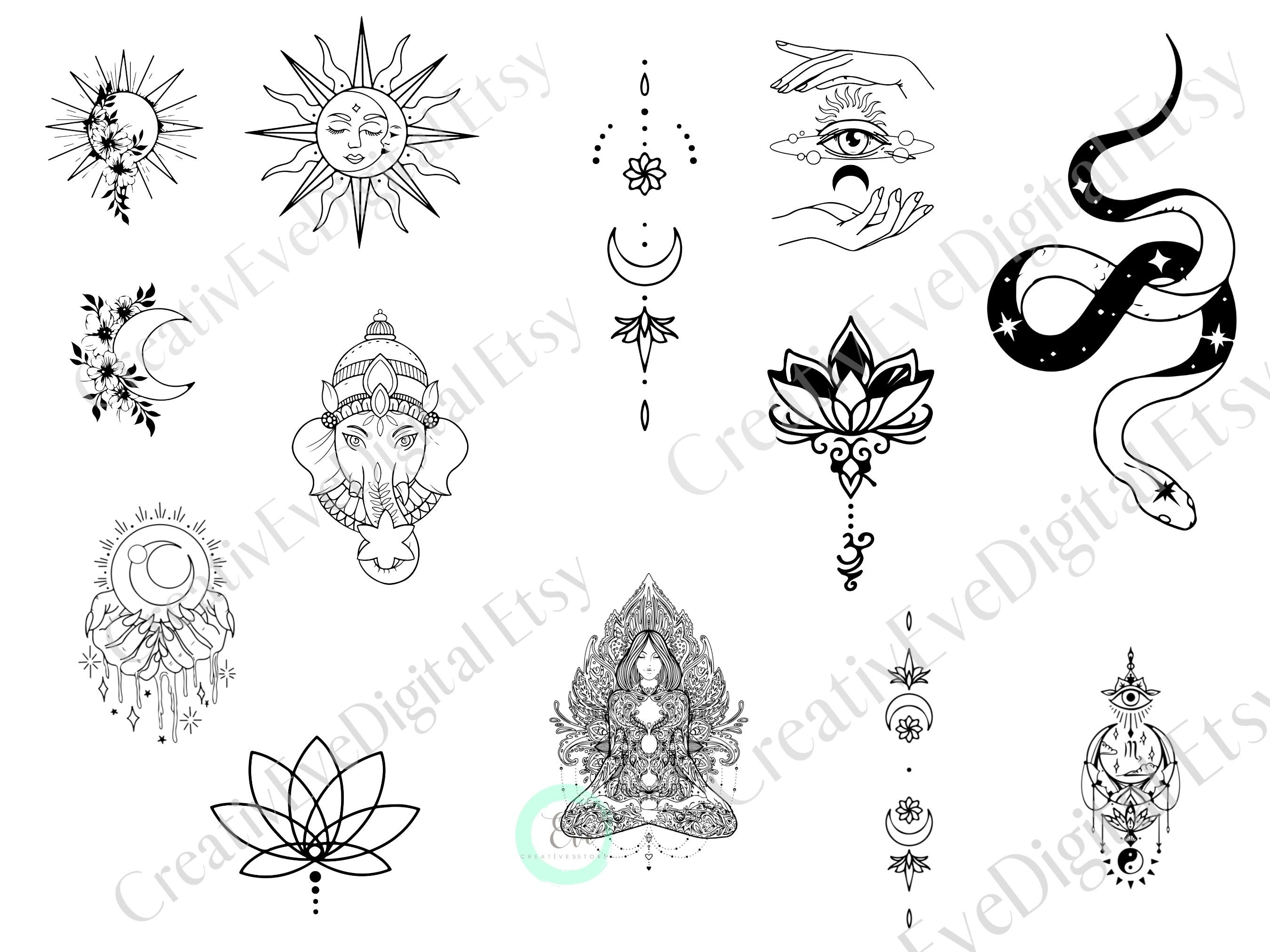The image showcases a collection of intricate, black-and-white astrological and spiritual-themed illustrations against a white background, all watermarked with the text "Creative Digital Etsy." These designs, likely available as downloadable PDFs on Etsy for use as stickers, tattoos, or other creative projects, vary in detail and subject matter. In the top left corner, there are several sunburst and sun motifs, and a moon adorned with flowers. Nearby, two hands holding a moon can be seen, followed by an elephant wearing a cap and featuring human-like eyes, holding a star. Further down, there is a flower and a central figure of a girl sitting cross-legged in a meditative pose with flowers behind her. Above her, another moon with flowers is depicted, flanked by two hands holding an orb with a crescent moon inside and dripping liquid. Other elements include an eye emitting rays with a small moon, numerous moon and floral designs, a lotus flower, and a snake adorned with stars. The overall composition is unified by its spiritual, mystical, and nature-inspired themes, all elegantly rendered in a cohesive monochromatic palette.